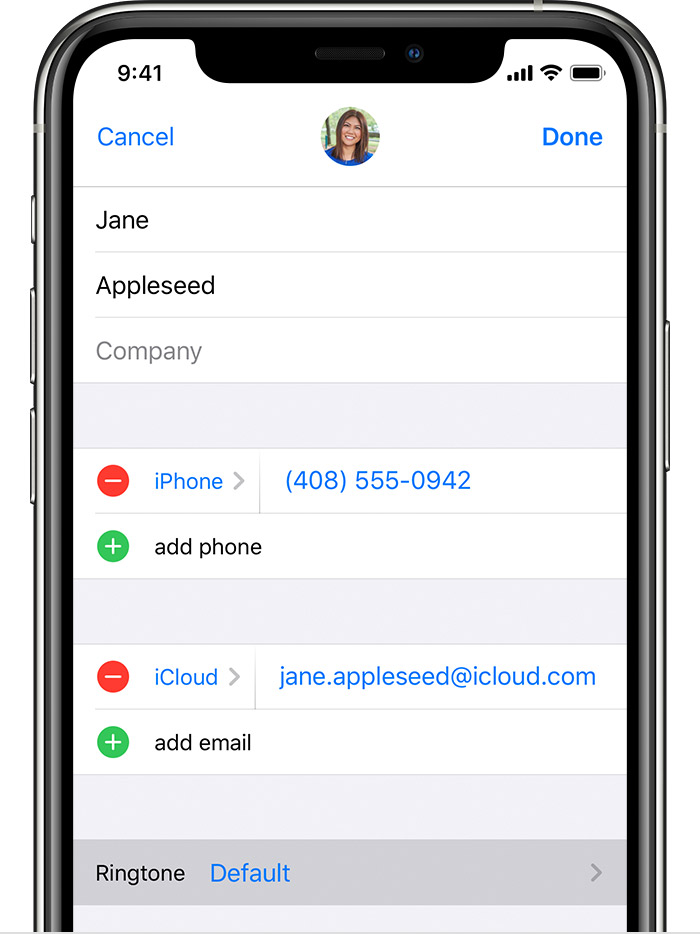Here’s the cleaned-up and detailed caption for the image:

“A screenshot of an iPhone contact for Jane Appleseed. Jane's profile picture shows a Caucasian woman with brown hair. The time displayed in the top-left corner of the screen is 9:41. The phone has full cellular reception with four bars, a strong Wi-Fi signal indicated by three out of three bars, and a fully charged battery.

Jane's contact details include a primary phone number with the area code 408 and the number 555-0942, displayed in blue text. There is an option to add a secondary phone number, marked by a green plus sign, but it has not been utilized.

Below the phone number is Jane’s iCloud email, jane.appleseed@icloud.com, also in blue text. There's a red minus sign next to the email, allowing users to remove it if necessary. An additional email can be added via a green plus sign, but no second email is currently listed.

Further down, there is an option to set or edit the ringtone for Jane’s contact. The ringtone is set to 'default,' displayed in blue text. Finally, in the top-right corner of the screen, there's a 'Done' button for when contact editing is completed.”